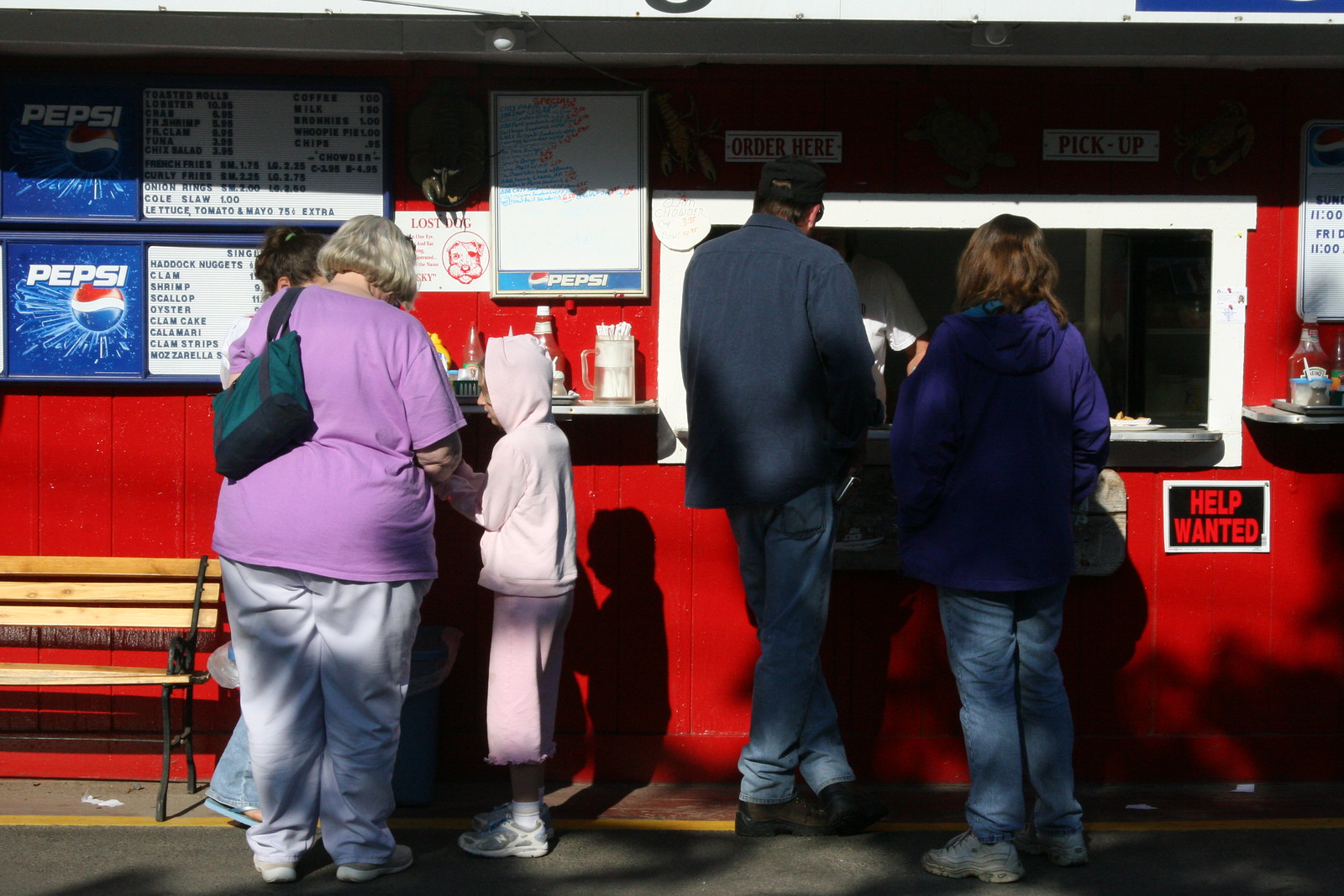In this detailed outdoor scene, we see a vibrant red concession stand bustling with activity as people loiter around its ordering and pick-up window. Positioned center-right is the main window, marked with "Order Here" and "Pick Up" signs. Below it is a help wanted notice. Immediately to the right of the window are a man in a blue shirt and jeans and a woman in a blue jacket and jeans, both at the ordering station.

To their left, a young woman, an older woman in a purple shirt with short bobbed gray hair, and a child dressed in pastel pink appear to be waiting for their order. The older woman's white pants are prominently visible, and she has her purse slung over her shoulder. Another group is seen to the far left, consisting of the backs of the older woman, her short gray hair clearly noticeable, and two other figures: a child wearing a hood and a sweatshirt, and a glimpse of another woman’s hair.

A large blue and white menu sponsored by Pepsi lists various seafood options like haddock nuggets, clam shrimp, scallops, oysters, and calamari. The menu is partially obstructed by the waiting patrons and sits above a condiment station with ketchup, mustard, and straws available for customers. To the far left of the image, there’s also a whiteboard likely used for specials, with a small "lost dog" sign beneath it. Finally, a brown bench positioned to the left provides additional seating for customers. The dynamic yet organized scene captures the lively atmosphere of this popular food stop.